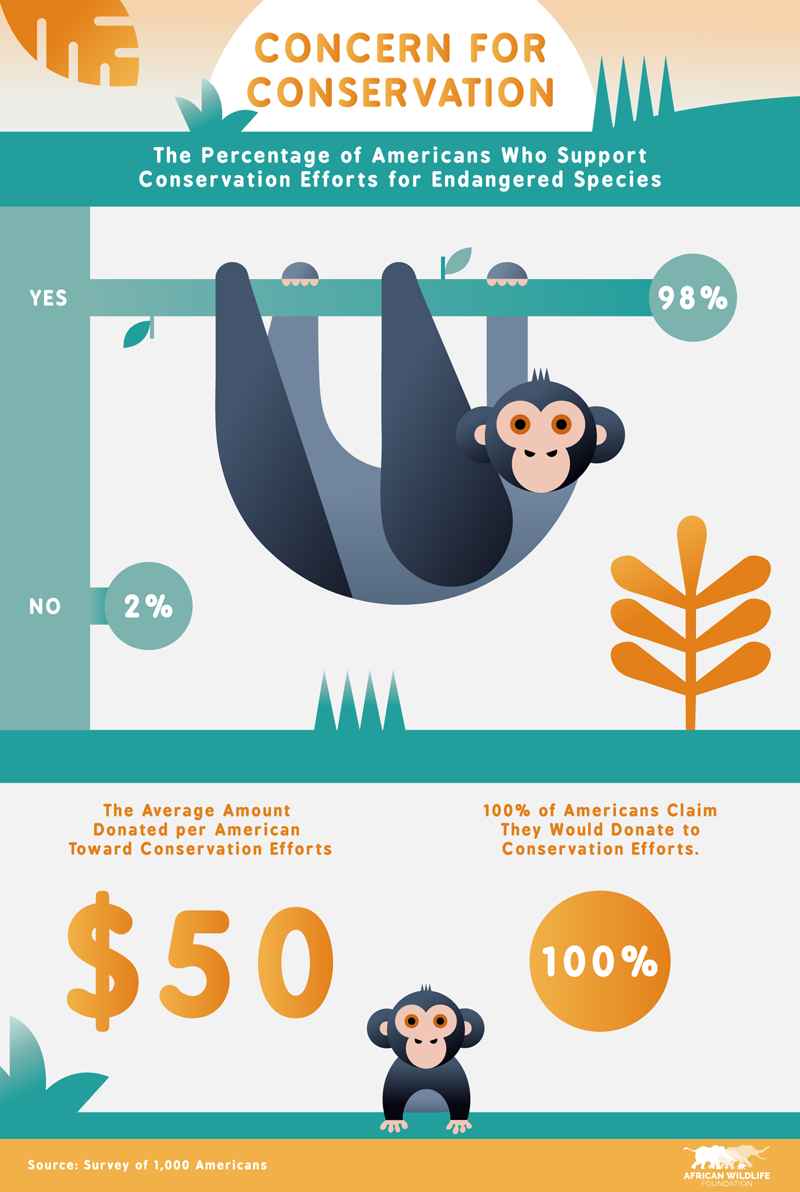The infographic, suitable for social media platforms like Facebook, features a detailed illustration on a white background with vibrant green and orange highlights. At the top, the title "Concern for Conservation" is prominently displayed in orange text above a half-sun graphic flanked by stylized trees and plants. An orange leaf icon adorns the top left corner.

The main body of the infographic contains text in white on green blocks, stating "The percentage of Americans who support conservation efforts for endangered species." The data is visually represented with a long horizontal line for "Yes" (98%), from which a cute monkey with circular ears, a tan face, and a black and gray body hangs. The shorter line for "No" (2%) is depicted similarly but without the monkey.

Beneath this, it says, "The average amount donated per American towards conservation efforts is $50" in an orange text block. To the right, it is noted that "100% of Americans claim they would donate to conservation efforts."

The bottom of the infographic features a source citation, "Source: Survey of 1,000 Americans," and the logo of the African Wildlife Foundation accompanied by an illustration of three elephants with an orange gradient. Additional details include a small monkey sitting on the ground with orange eyes and a green bush with three leaves to the left of the monkey.